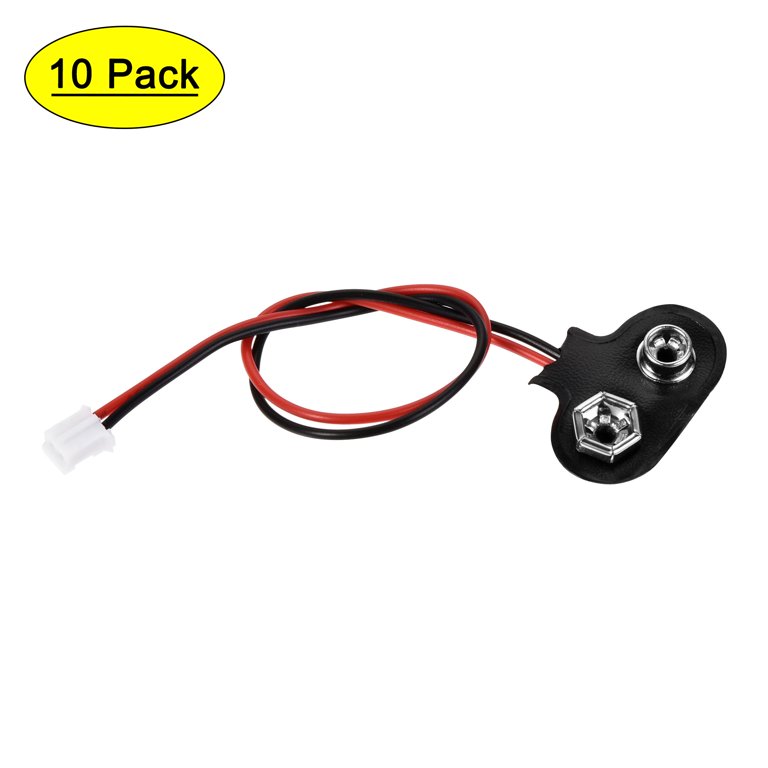The product photograph features a top-down view of a small wired device designed for connecting to a 9-volt battery. At the top left of the image, a yellow oval outlined in black displays the underlined text "10-pack" in bold black letters, set against a bright white background suggesting it is a display picture for online sales. 

The device itself showcases a pair of silver ports: a circular metal port and a hexagonal port, both securely fastened to a black oval leather pad. This pad is connected to two wires, one red and one black, which are loosely knotted together for easy separation. At the end of these wires, a white plastic wire cap provides a neat finish and additional protection. The detailed layout and the simplicity of the components indicate this is a well-designed, user-friendly product designed for ease of connection and secure attachment to a 9-volt battery.